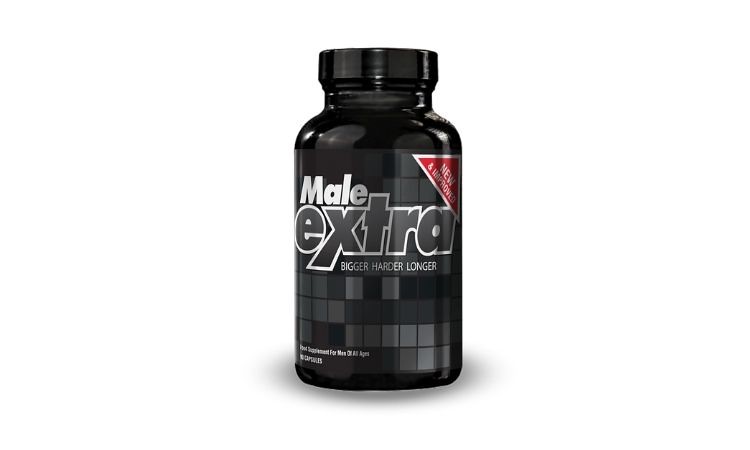A black bottle containing a male vitamin supplement is adorned with a sleek label featuring a color scheme of black, gray, and silver. In the top right corner, a red triangle with silver text declares "NEW AND IMPROVED." The bottle is secured with a black screw-on lid. The label displays the word "male" in bold white letters at the top, followed by "extra rodent" in lower-case gray letters outlined in silver. Below that, the phrase "BIGGER, HARDER, LONGER" stands out in all capital silver letters. In the bottom left corner of the label, the text mentions the supplement being suitable "for men of all ages," though the exact number of capsules is obscured. The background of the label is patterned with scattered gray squares.